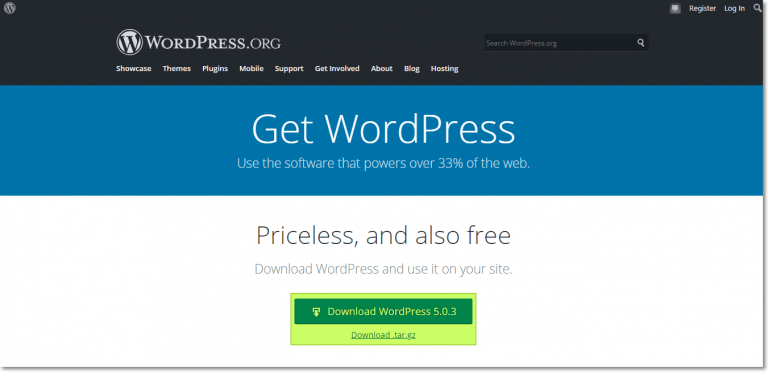The image displays a snapshot of the WordPress.org homepage. At the top, there is a black rectangular header containing the WordPress logo—a "W" enclosed in a circle—and several menu options including "Showcase," "Themes," "Plugins," "Mobile Support," "Get Involved," "About," "Blog," and "Hosting." To the right of these options, there is a search bar labeled "searchwordpress.org," a registration link, and a login link.

Below the header, there is a bluish-teal section that prominently features a call-to-action message: "Get WordPress." The text highlights that WordPress powers over 33% of the web and is both "priceless" and "free." This section encourages users to download and use WordPress on their own websites.

Further down, the background shifts to white. In this area, the page provides information about downloading WordPress, specifically version 5.0.3. A bright fluorescent green box with a darker green "Download WordPress" button stands out at the bottom, offering the download in .tar.gz format.